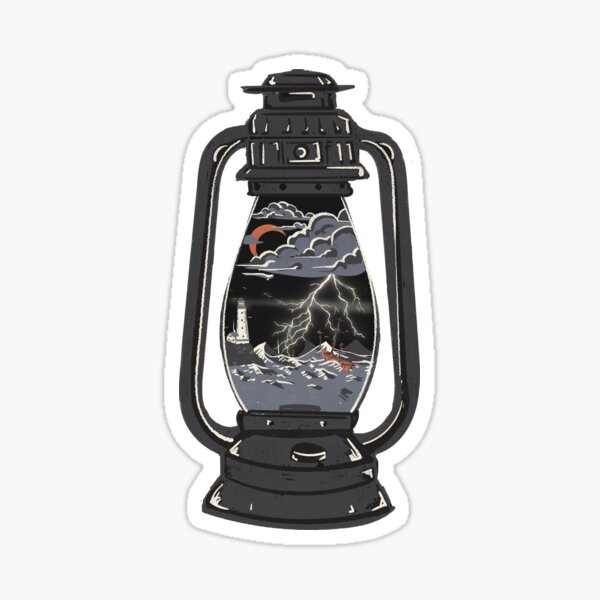The image showcases a camping lantern set against a complete white background, with a subtle border and shadow giving it a sticker-like appearance. This gunmetal gray lantern, which appears to have a handle on both sides and a lid-like top, has an oval-shaped body with cut-off top and bottom parts. 

Within the glass of the lantern is an elaborate, monochromatic artwork that tells an intense story. In the upper left, a crescent moon curves towards a dark, stormy sky, where lightning bolts streak through gray clouds. Below, a tumultuous ocean is depicted in dark gray hues, with waves resembling a violent sea. A lighthouse stands in the background, seemingly on the edge of an island, while what might be a ship in distress appears with hints of red suggesting flames or damage. The intricate scene offers a stark contrast to the typical light you'd expect to see inside a lantern. 

At the center of the lantern's body, there's a knob or button likely intended to turn the light on and off, though the focus is undoubtedly on the dramatic image within.